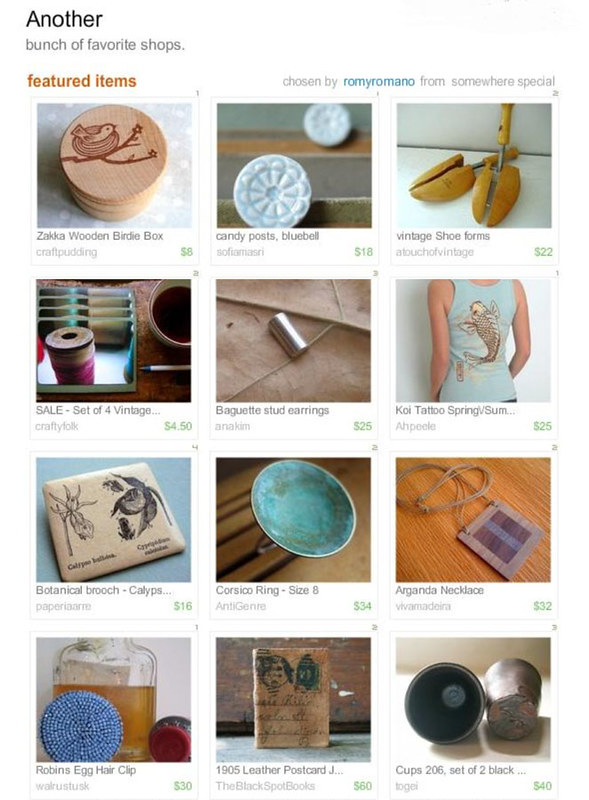The image showcases a screen capture of an Etsy-like online shop featuring a curated selection of 12 handmade and vintage items. The background is white, and the layout is organized into a grid with three columns and four rows. At the top of the image, a black title reads "Another Bunch of Favorite Items," followed by an orange subtitle "Featured Items Chosen by Romy Romano from Somewhere Special," with Romy's name highlighted in light blue.

Each item is presented within its own box, accompanied by distinctive captions and prices marked in green. The items on display encompass various household and arts-and-crafts goods. For example, the top row includes a "Zaka Wooden Birdie Box," followed by a "Sale Set of 4 Vintage Spools of Thread," and a "Botanical Brooch" adorned with insect designs. The next items include a "Robin's Egg Hair Clip" with blue beads and "Candy Post Bluebell."

In the center column, you will find a "Banquet Stud Earrings," a "Corsica Ring Size 8," and "1905 Leather Postcards." Moving to the right column, it features "Vintage Shoe Forms," a "Koi Tattoo Spring/Summer," an "Arganda Necklace," and a "Cups 206 Set of 2 in Black."

The overall color scheme includes hues of blue, orange, and black, giving a vibrant yet rustic feel, which is complemented by the burlap color elements within the product images. The detailed presentation highlights each item's unique characteristics and appeal, making it easy for potential buyers to explore and appreciate each product.